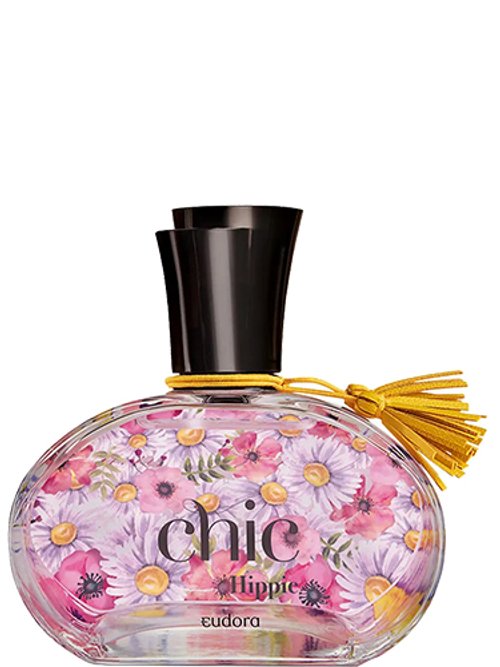This image features a bottle of women's perfume set against a completely white background, devoid of any other elements. The transparent glass bottle has an oval shape and gives the impression of being heavy and sturdy. Its black cap sits firmly on top, under which is a yellow fringe tassel to the right side, adding a touch of bohemian elegance. The bottle is labeled "Chic Hippie" by the manufacturer Eudora, spelled out in black text. It's adorned with vibrant, detailed floral designs, including large pink peonies with black centers and pink-lavender daisies with gold centers. The flowers are intricately illustrated, with additional hues of purple, yellow, green, and dark purple, contributing to its colorful and eye-catching appearance. The image has a professional quality, resembling a stock photo typically used in advertisements, emphasizing the perfume as a desirable product for sale.